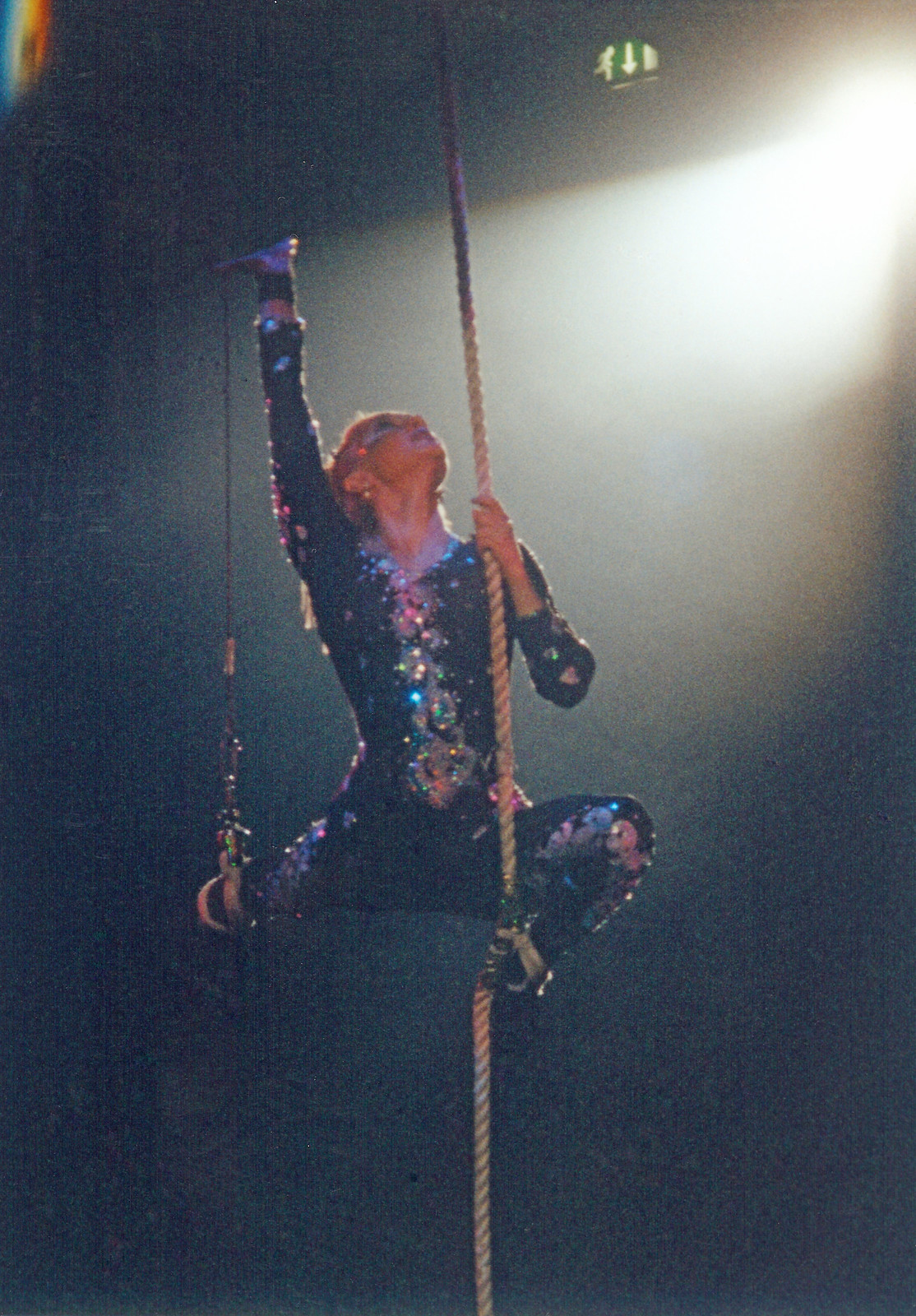The image is a grainy, vintage photograph that appears to be from a magazine or newspaper, showcasing a circus performer mid-act. The performer is a woman wearing a skin-tight, dark leotard, likely black or dark green, adorned with sequins that create a sparkling effect under the spotlight. Her costume features sparkling decorations that are concentrated on the chest, knees, and cuffs, giving it a jewel-like appearance. She is suspended upright on a thick rope wrapped around one leg, with her other leg and one arm also engaged with the rope, indicating she is in the midst of an acrobatic maneuver. Her head is tilted upwards, accentuated by makeup around her eyes and mouth, adding to the theatrical element emphasized by the dramatic lighting. The background is mostly dark, save for a spotlight that illuminates her, and a green sign with a human figure and an arrow pointing downward can be seen at the top of the image.